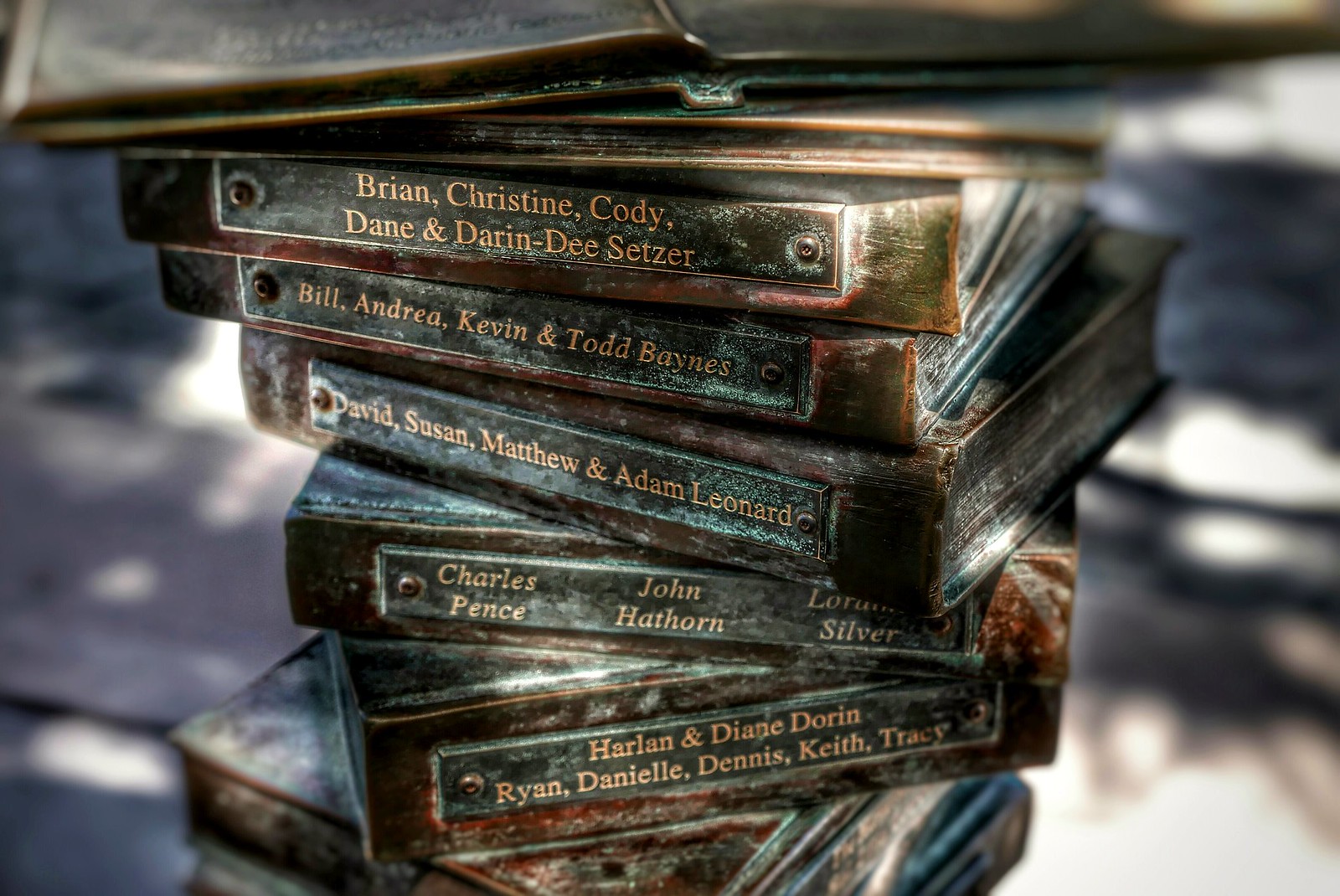In the image, there is a haphazard stack of very old and dusty, tattered brown books or photo albums. They are not neatly arranged; some are crooked, slanted, and twisted. Mold, including patches of green mold, is visible on the albums, primarily on the inserts and plaques that label each book. The background is a gray-black blur, emphasizing the decayed objects. The open book sits at the very top, and the titles listed on the spines of the books below it are in various colored texts, including orange and black. The labels include names such as:

- **Top book (open)**: Unspecified names due to it being open.
- **Next book**: Brian, Christine, Cody, Dane, Darren D. Setzer.
- **Below that**: Bill, Andrea, Kevin, and Todd Baines.
- **Next**: David, Susan, Matthew, and Adam Leonard.
- **Following**: Charles Pence, John Hathorne, and Lorraine Silver.
- **Bottom (where the seam is)**: Harlan and Deanne Doran, Ryan, Danielle, Dennis, Keith, Tracy.

The collection, numbering seven in total, suggests a rich, albeit neglected, history encased within these deteriorating volumes.